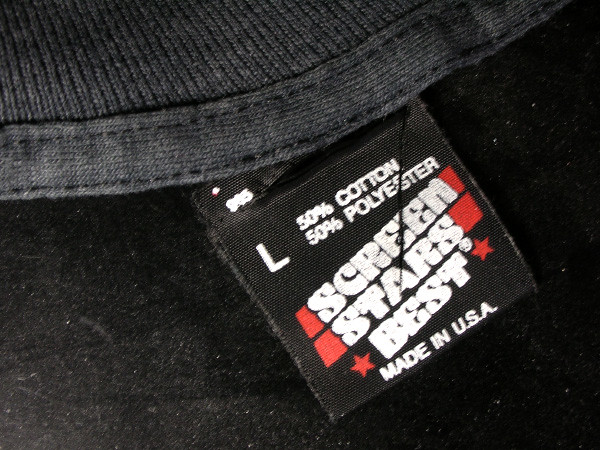In this photograph, we see a close-up view of the inside tag of a black t-shirt, meticulously stitched to the collar. The collar's slight curve highlights the stretchy nature of the fabric. The tag itself is a black square adorned with white text that reads: "L. 50% cotton, 50% polyester. Screen starts best. Made in USA." Notably, the words "best" are flanked by two small red stars, adding a touch of color to the otherwise monochromatic label. It’s evident that the tag is starting to come unstitched from the hem, with a few threads hanging loosely, suggesting some wear and tear.